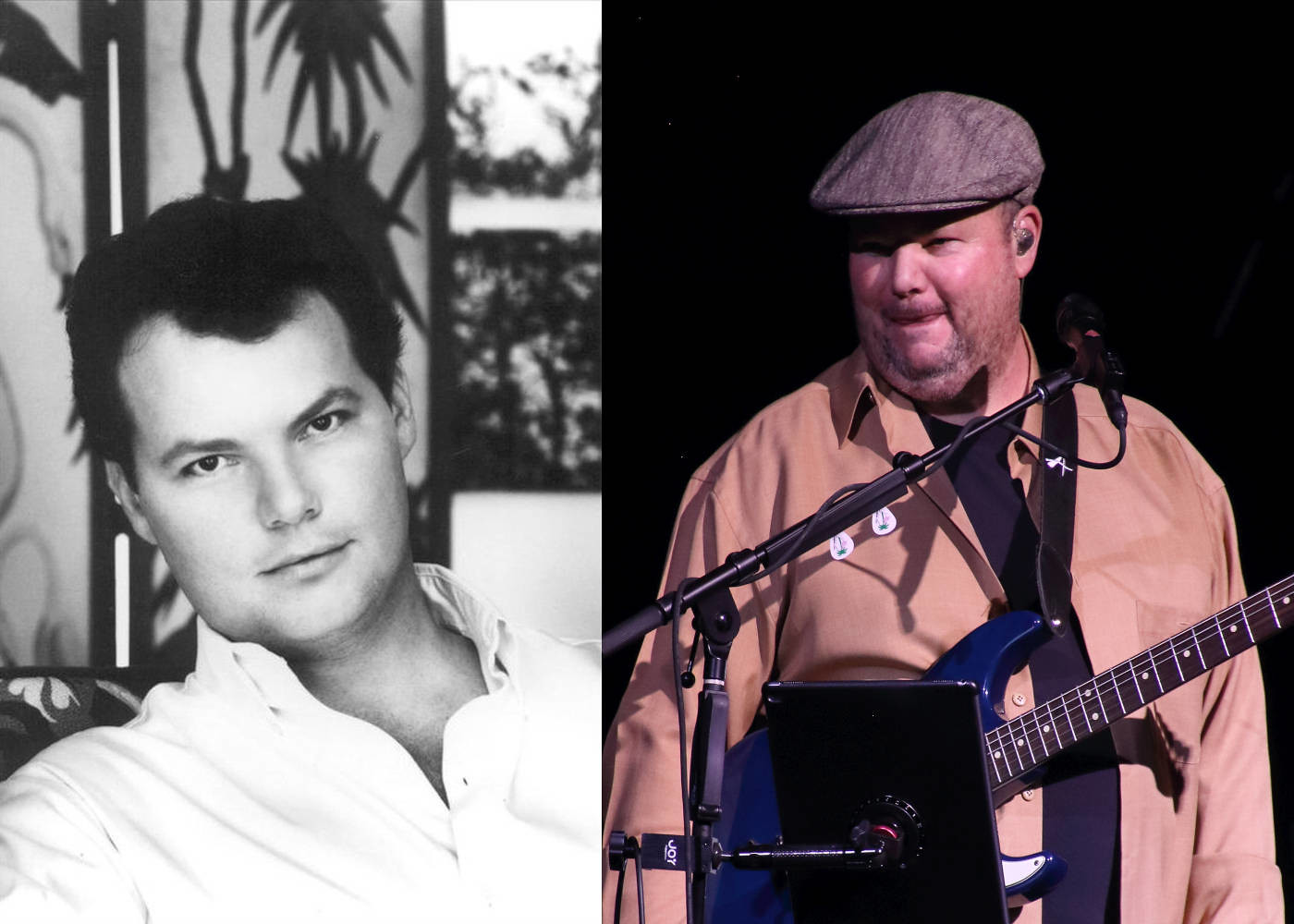The composite image consists of two photographs of Christopher Cross, juxtaposed to highlight the passage of time. The left image, in black and white, captures a younger Cross with dark hair, dark eyes, and dark eyebrows. Dressed in a white button-up shirt, he gazes directly at the camera, set against what appears to be an indoor scene with a decorative divider and visible shrubbery through an opening. The right image, in full color, shows a much older Cross. He wears a gray cap and has a fuller face with thin facial hair, including stubble and a double chin. His outfit consists of a beige rose-colored long-sleeve button-up shirt, open at the collar, with a black shirt underneath. Holding a blue electric guitar on a strap across his shoulders, Cross is seen with a microphone positioned near his mouth, and an iPad or similar device on a stand in front of him. The background in this image is stark black, emphasizing his current stage setup.